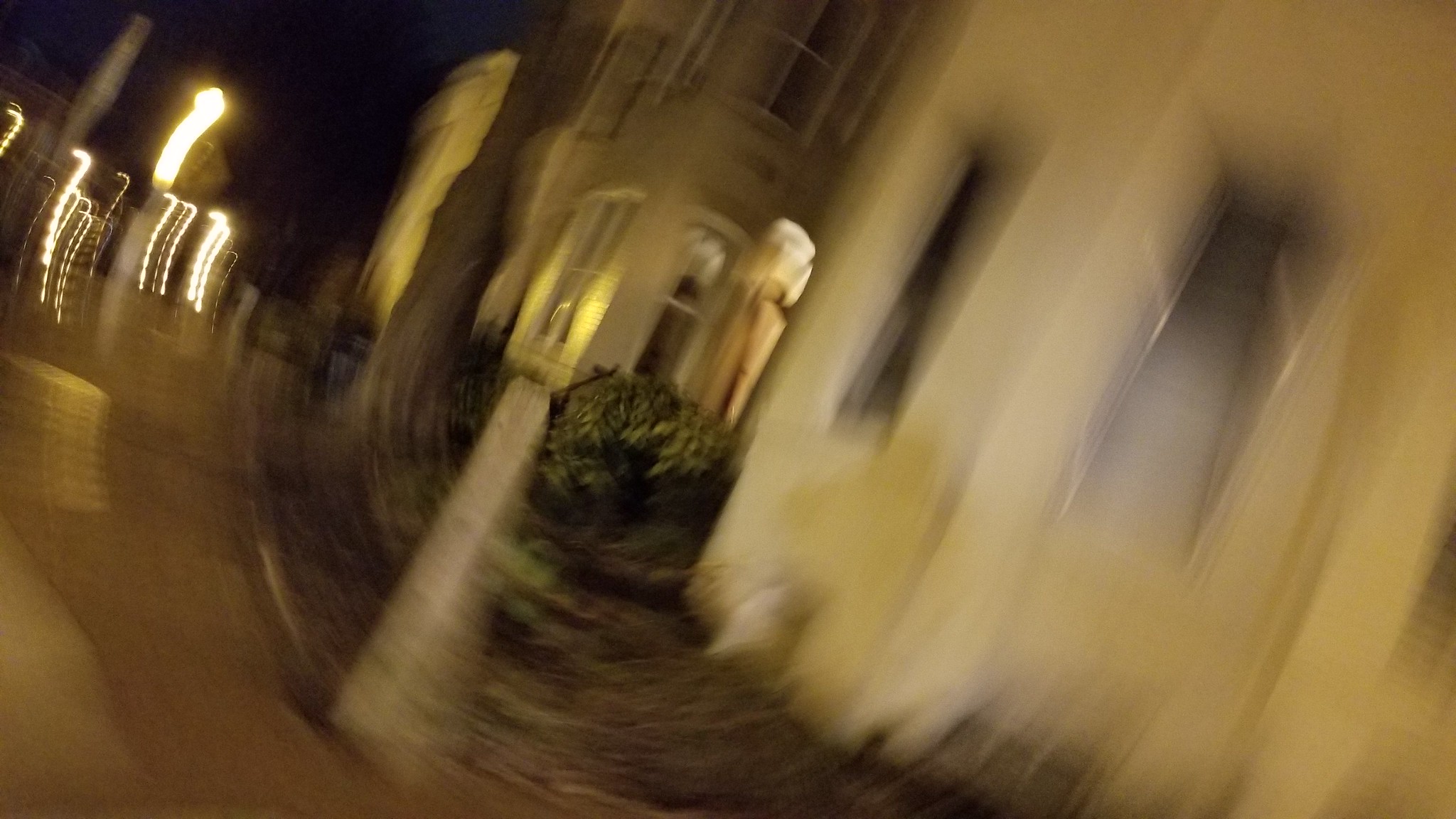The image depicts an extremely blurry nighttime scene with a distinct circular motion blur pattern, suggesting intentional movement during the capture. At the center of the image, there is a white-rimmed window with white molding, adorned with a white curtain, and a green bush situated below it. This window is positioned on the right-hand side, part of a white building that appears old. To the left of this building, another white building can be seen, with a sidewalk or road running alongside. There are streetlights towards the upper left corner, reflecting off the windows and sides of the buildings, adding a whitish-yellowish glow to the scene. The rest of the image is a swirling blur, creating an impression of two or more large buildings and possibly a small tower or statue amidst this motion. The overall atmosphere is dark, with the sky in the upper left corner appearing black. The central clarity of the window and bush contrasts sharply with the surrounding blur, emphasizing the static amidst the dynamic.